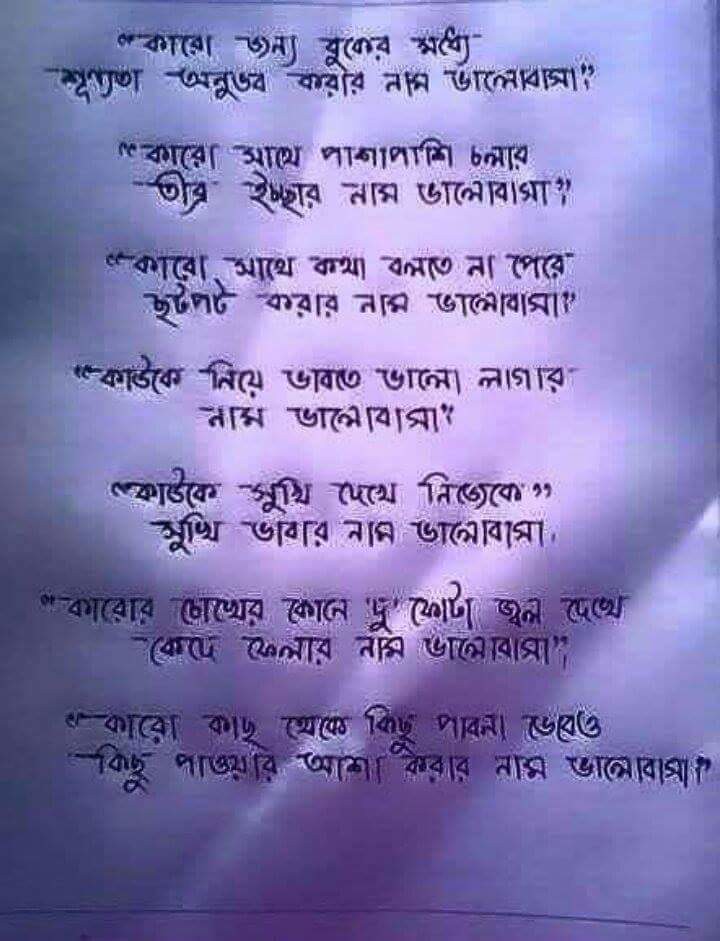This image displays a well-lit piece of white paper which appears to have a light blue hue, possibly due to shadows or the ambient lighting. The paper has a slightly wrinkled texture, suggesting it has been folded in a few spots. The paper contains lines of foreign writing, which appear to be upside down. 

The layout consists of several sections: an initial two lines followed by a space, then another two lines, and this pattern repeats with intermittent spaces, leading to a total of around 14 lines. The characters in the writing do not resemble typical English or oriental scripts. They seem detailed with a mix of straight and curved lines, and though they are perceived as letters, their complexity makes them unfamiliar to someone used to the English language.

The background of the image features wispy white clouds on a light blue sky, adding an artistic element. The lower right part of the image especially shows a light blue color, merging with streaks of clouds. This setting adds a tranquil and serene contrast to the intricate and somewhat mysterious foreign script on the paper.